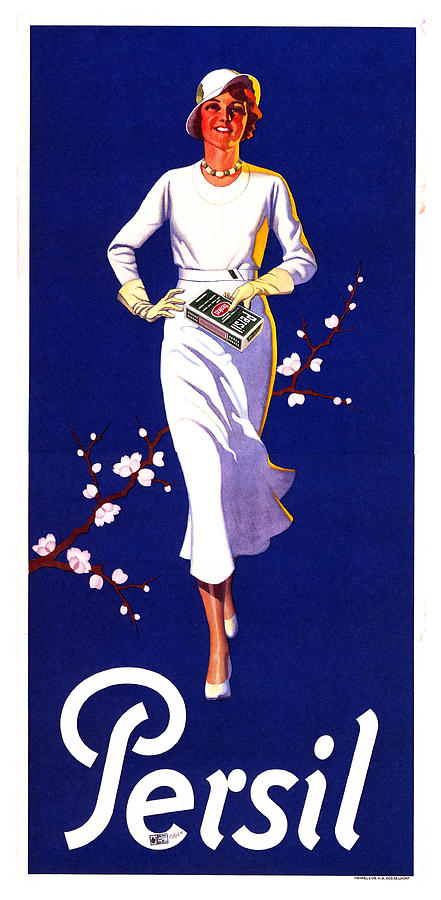This vertically aligned, retro-style advertisement appears to be from the 1930s or 40s, featuring an elegant woman in an animated graphic style. The background is a solid dark blue, which makes the figure stand out strikingly. The woman is depicted walking gracefully, with her right foot poised in front of her left. She is wearing a long-sleeve white dress that flares out towards the bottom, creating a sense of fluid motion. A belt cinches the waist of her dress, highlighting her slender figure. She pairs this with white high heels, a necklace, and pale yellow (or beige) gloves. On her head, she dons a white tilted hat that frames her short red (or possibly brown) hair. She carries a box labeled "Persil" in white text. The same name, "Persil," is prominently displayed at the bottom of the image in large, curved white letters. Behind her, a brown tree branch adorned with white flowers, tinged with pink, sweeps diagonally across the blue background, adding a touch of natural elegance to the advertisement. The overall impression is of a sophisticated, vintage advertisement, likely for a product such as detergent.